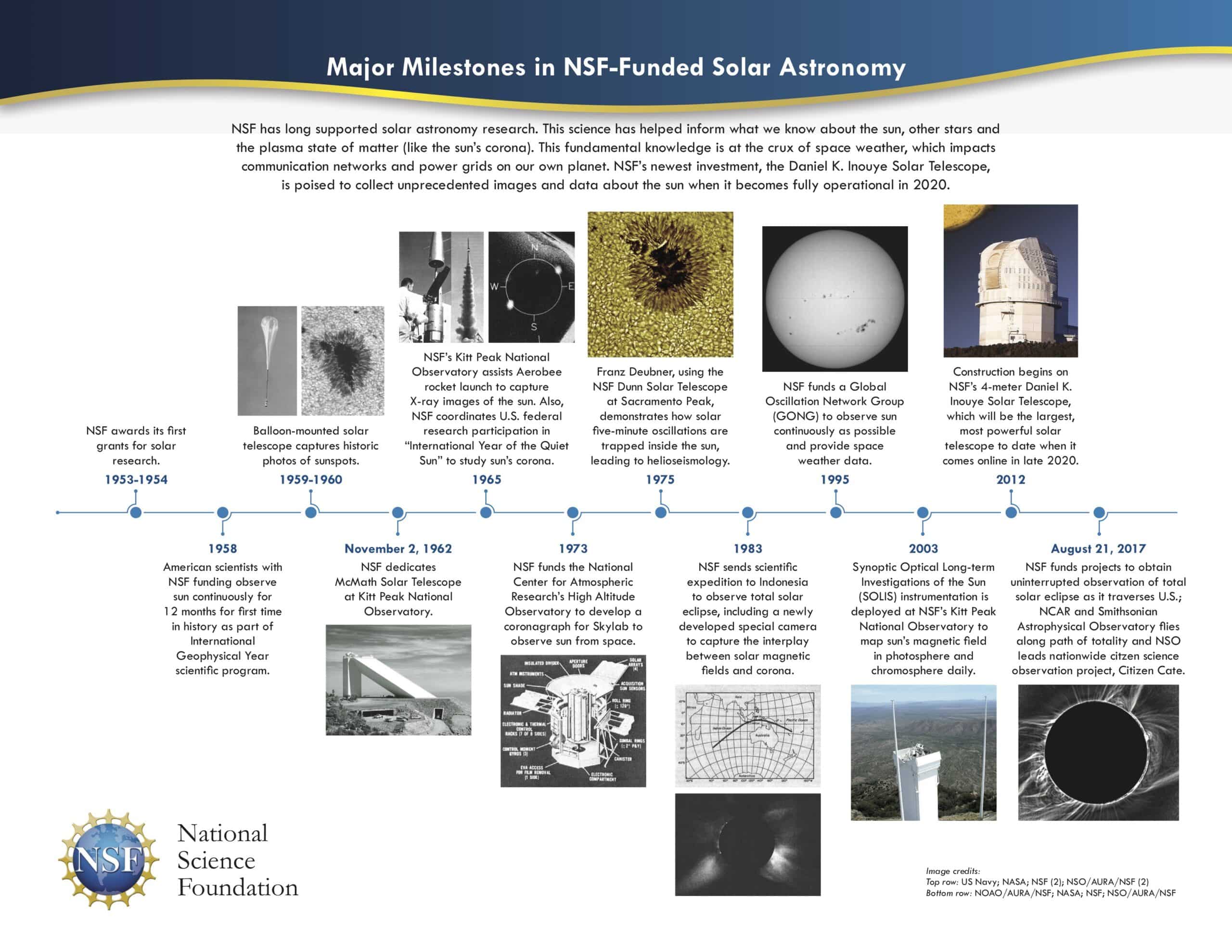This detailed poster, produced by the National Science Foundation (NSF), presents a comprehensive timeline titled "Major Milestones in NSF-Funded Solar Astronomy." The poster, primarily white with a blue top border, charts the significant developments in solar astronomy from 1953 to 2017. At the top, in white text against the blue background, it introduces the topic, explaining that NSF has long supported solar astronomical research—contributing substantially to our understanding of the Sun, other stars, and plasma states like the Sun's corona. This research is crucial for understanding space weather, which affects Earth's communication networks and power grids.

A blue horizontal line traverses the white background, marking significant dates with black text descriptions and images below each dot on the timeline. The timeline starts in 1953 when NSF awarded its first grants for solar research, then highlights key advancements such as the historic balloon-mounted solar telescope photos of sunspots in 1959-1960. It also marks the NSF-funded National Center for Atmospheric Research's development of a coronagraph for Skylab in 1973 and notes the commencement of the Daniel K. Inouye Solar Telescope construction in 2012.

In the bottom left corner, the NSF logo, a blue globe symbolizing Earth with white NSF letters, is accompanied by the text "National Science Foundation" in black. The poster includes eleven significant events, most illustrated with images (predominantly black and white with hints of yellow), like a balloon, a sunspot, and a solar telescope, depicting the evolution and milestones in solar astronomy funded by NSF.